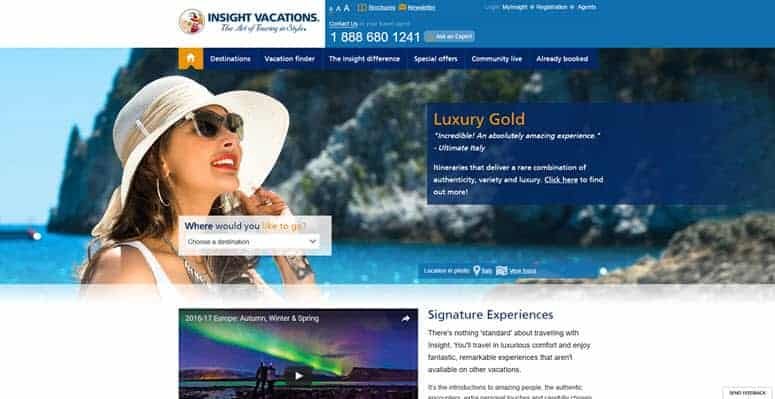The image is a screenshot of a vacation website called "Insight Vacations," characterized by a clean white and blue color scheme. Dominating the center of the page is a woman epitomizing a vacation vibe; she wears a wide-brimmed sun hat, primarily white with a beige stripe at the top. Complementing her look, she dons brown sunglasses with silver rims and light lipstick. The woman's expression is one of awe and amazement as she gazes upward and to the right, her mouth slightly open and her left hand thoughtfully placed on her chin.

Above her, in the top left corner, is the website's title, while the top right corner displays a contact number: 1-888-680-1241. To the right of the woman, the words "Luxury Gold" stand out in blue text, accompanied by quotations that describe the experience as "Incredible and absolutely amazing." Additionally, there is a reference to a package called "Ultimate Italy." The overall aesthetic and content make it clear that this site offers curated luxury vacation packages.